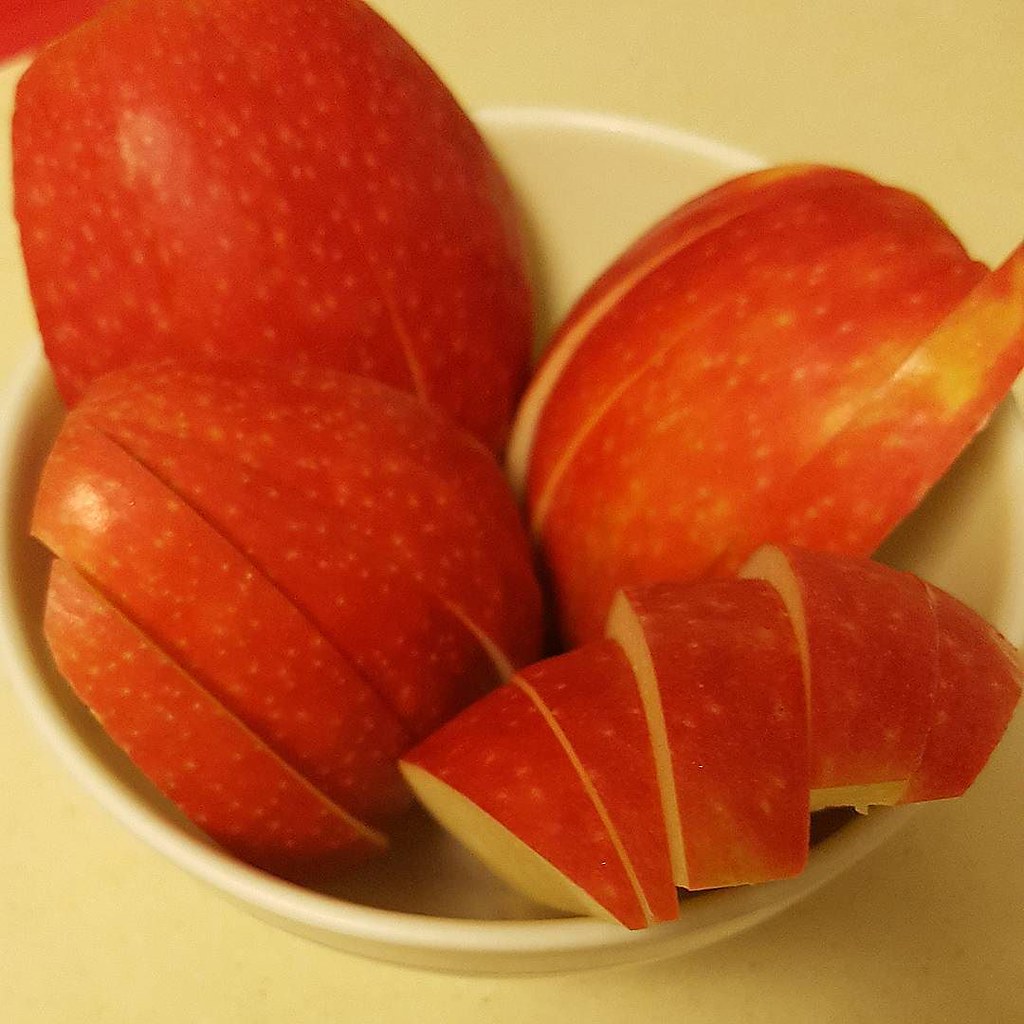The image is a square color photograph taken under artificial lighting, giving it a warm, yellowish tungsten hue. The photograph is a close-up shot, showing a small off-white ceramic bowl placed on what appears to be a yellow surface. Inside the bowl, there are several red apples that have been cut into thin slices. The slices are arranged into four distinct sections or quadrants, with their inner, sliced portions facing the viewer and their outer skins touching each other within the bowl. In the upper left corner of the bowl, there is a section that may be a half apple, appearing not to be sliced. The apples exhibit a pinkish-orange tint with small light green specks dispersed throughout their flesh, suggesting they were sliced with precision. The image allows a top-down view, clearly displaying the textures and arrangement of the apple slices.